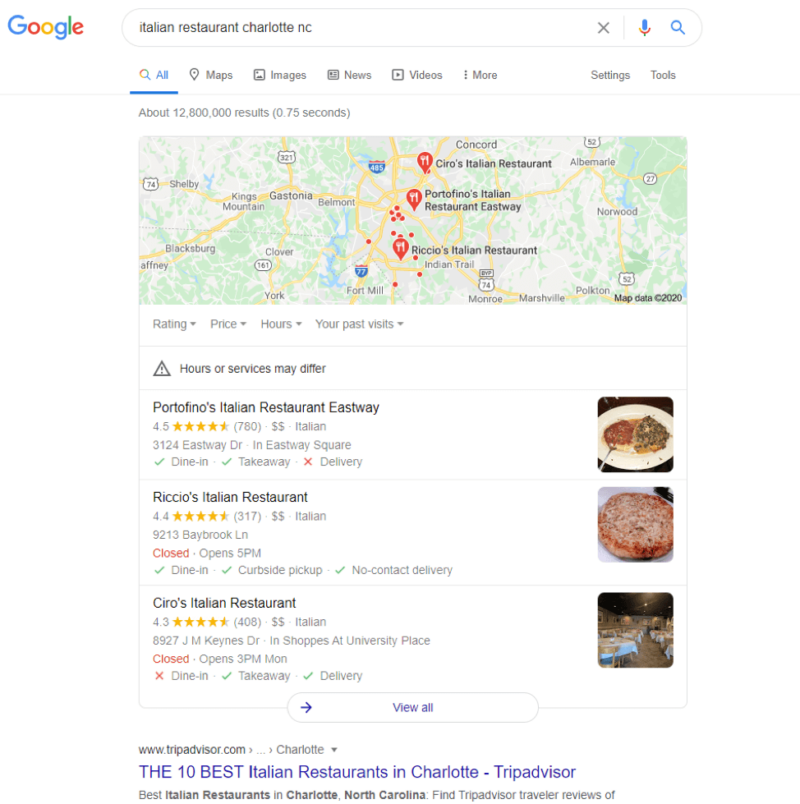The image displays a Google search results page. On the top left, the colorful Google logo is prominently visible in blue, red, orange, and green. Adjacent to the logo is the search bar containing the query "Italian restaurants Charlotte NC" in black text. In the top right corner, there is an "X" icon, followed by a microphone icon and a magnifying glass icon representing the search button.

Below the search bar, there are several navigation options labeled from left to right: All, Maps, Images, News, Videos, More. To the far right are Settings and Tools options. Underneath these options, the page indicates that there are about 12 million results found within 0.75 seconds.

Following this information, a map is displayed, featuring various green areas interspersed with white spaces and yellow roads, intricately weaving like a maze. Highlighted points on the map indicate the locations of Italian restaurants, with several key points labeled: Ciro's Italian Restaurant, Portofino's Italian Restaurant Eastway, and Riccio's Italian Restaurant. Each location is marked with a red pinpoint icon.

Directly below the map, there are dropdown menus labeled Ratings, Price, Hours, and Your Past Visits. A note mentions that hours and services may differ. Below this, there are three distinct search results:

1. Portofino's Italian Restaurant Eastway
2. Riccio's Italian Restaurant
3. Ciro's Italian Restaurant

Each restaurant listing includes a rating out of five stars, with scores of 4.5, 4.4, and 4.3, represented by gold-colored stars. To the right of each listing, images are provided: plates of food, which may include beet loaf or pizzas, and dining room settings. At the bottom center, a white button with blue text invites users to "View All."

Further down, there is another search result from TripAdvisor.com, labeled "The 10 Best Italian Restaurants in Charlotte - Trip Advisor." Below this, in black text, is a brief description summarizing TripAdvisor traveler reviews for the best Italian restaurants in Charlotte, North Carolina.

The entire page features a clean, white background, maintaining Google’s signature minimalistic design.